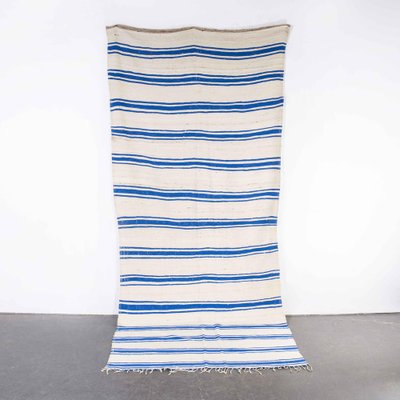This image features a close-up shot of a long, rectangular rug or towel, predominantly white with a pattern of blue stripes. The stripes are arranged in a sequence of a thin blue line, followed by a thick blue stripe in the middle, and then another thin blue line, repeating throughout the length of the fabric. There are 15 stripes in total. The material, made of fabric, is mounted vertically on a white wall, likely fastened at the corners, and extends downward, lying smoothly onto a gray, slate-type concrete floor. The bottom edge of the rug is adorned with white tassels that rest on the floor. The setting is minimalistic with no additional features other than the stark white wall and the gray flooring.